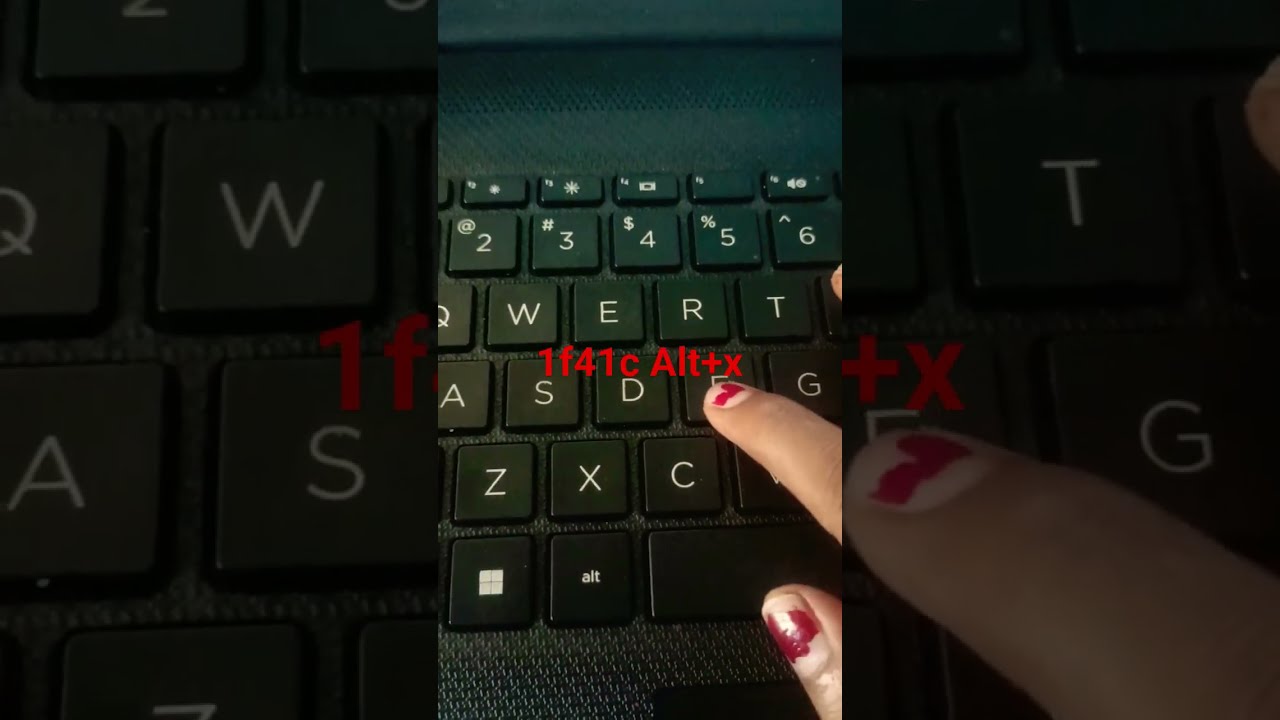The image is a close-up photograph of a black QWERTY keyboard, specifically focused on the region spanning from the A key to the G key. Prominently featured is a person's right forefinger, adorned with chipped red nail polish, pressing the F key. The keyboard keys are black with light gray or white lettering. Overlaying the central image is red text that reads "1F4 1C ALT + X," with the letter "A" capitalized. Flanking the photograph on both sides are vertical strips that present a darkened, zoomed-in version of the same keyboard image, enhancing the portrait orientation of the overall composition.